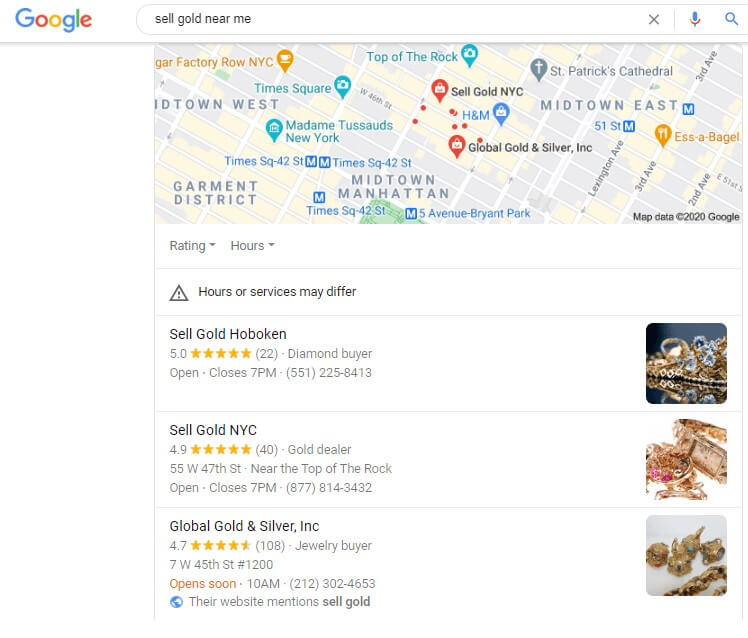This image appears to be a screenshot of a Google search results page. The background is predominantly white with the Google logo featured prominently in the top left corner. Next to the logo is a search bar that contains the query "sell gold near me," accompanied by an 'X' icon to clear the text, a microphone icon for voice input, and a search icon. 

Below the search bar is a Google Maps widget displaying a section of Manhattan, New York City. The map is enclosed in a rectangular frame and highlights various types of businesses, such as churches and restaurants. Notable points marked on the map include Midtown Manhattan and Madame Tussauds New York. Specific locations related to selling gold are also listed, such as "Sell Gold New NYC" and "Global Gold and Silver Inc."

Beneath the map are dropdown menus for ratings and operating hours. A caution symbol with an exclamation point warns that hours or services may differ. Following this warning, the screenshot lists three nearby places where gold can be sold:
1. Sell Gold Hoboken
2. Sell Gold NYC
3. Global Gold and Silver Inc.

Each listing is accompanied by an image of jewelry to the right, adding visual context to the search results.